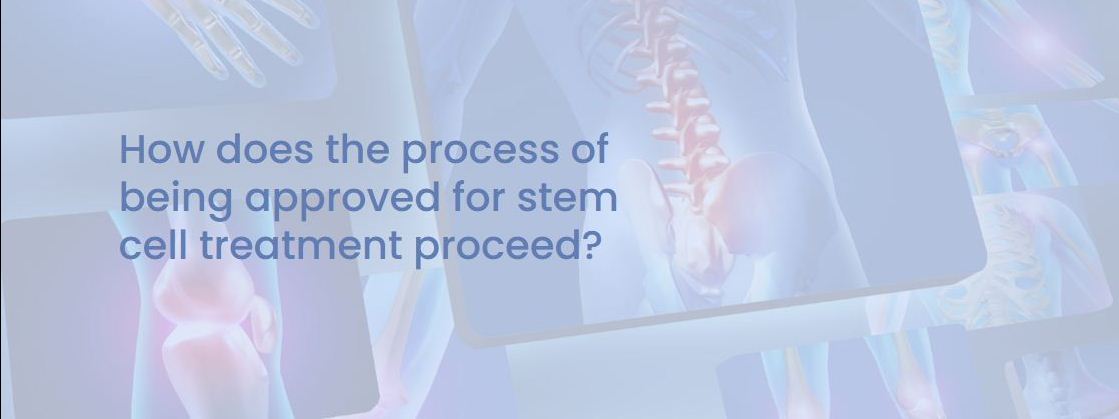The image depicted is reminiscent of a PowerPoint slide or possibly an informational poster. It has an elongated and narrow layout with a background featuring a collage of x-ray-like images displaying various skeletal structures. These images have a faded blue tint, with bones highlighted in shades of pink, red, and purple. Prominently, the central image shows a spine, emphasizing the vertebrae, ribcage, and hip bones in red. Flanking the central image are partial x-rays of knees and additional skeletal sections, also highlighted in red. The content of the slide is minimal, consisting of a succinct question in blue sans serif font, aligned to the left. It reads: "How does the process of being approved for stem cell treatment proceed?" The focus is clearly on the text, which spans three lines and ends with a question mark. This composition, with its medical imagery and straightforward question, suggests an educational context, likely providing an overview of the stem cell treatment approval process.